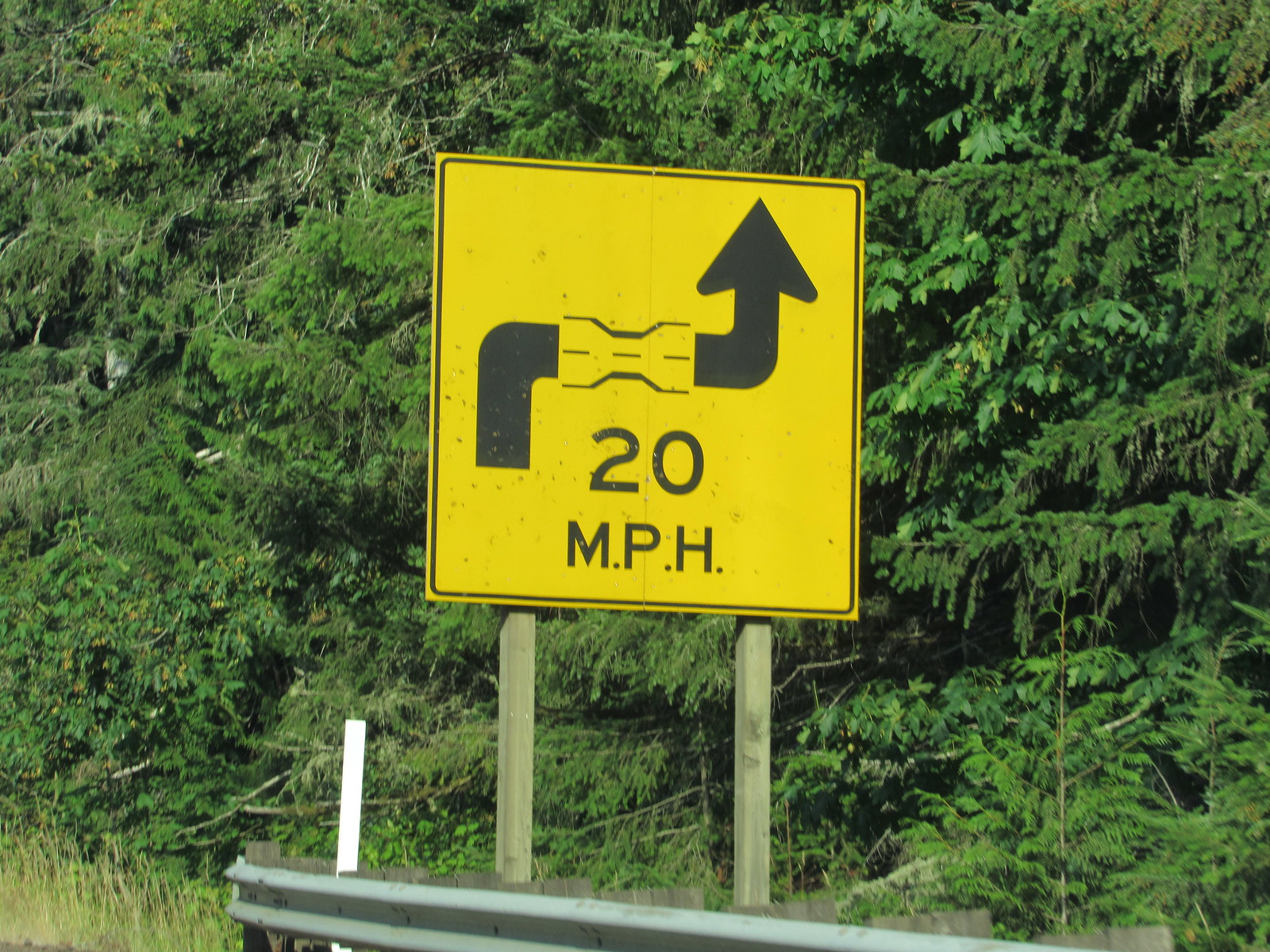This image captures a close-up of a road sign set against a dense backdrop of vibrant, evergreen trees, indicating a forested area. The trees are closely packed, rendering an almost impenetrable green canopy, while a few dead, bare branches on the left-hand side add a touch of variation to the scenery. The setting is bright and illuminated by ample sunshine, creating a picturesque landscape. 

In the foreground, a metal guardrail extends horizontally, partly obscuring the base of the sign and accompanied by a patch of green grass to its left. The road sign is mounted on sturdy gray metal posts, two in number, providing stability against the natural backdrop. The nearly square, yellow road sign features intricate black lettering and symbols. It reads "20 M.P.H." and graphically illustrates the road's trajectory and changing conditions. Starting from the left, the road ascends straight before a brief right-hand turn. This is followed by an indication that the road narrows from two lanes to one before widening back into two lanes, with a final sharp left turn depicted by a black arrow. This detailed sign assists drivers in anticipating the upcoming road dynamics, ensuring a safe journey through this beautiful, forested area.